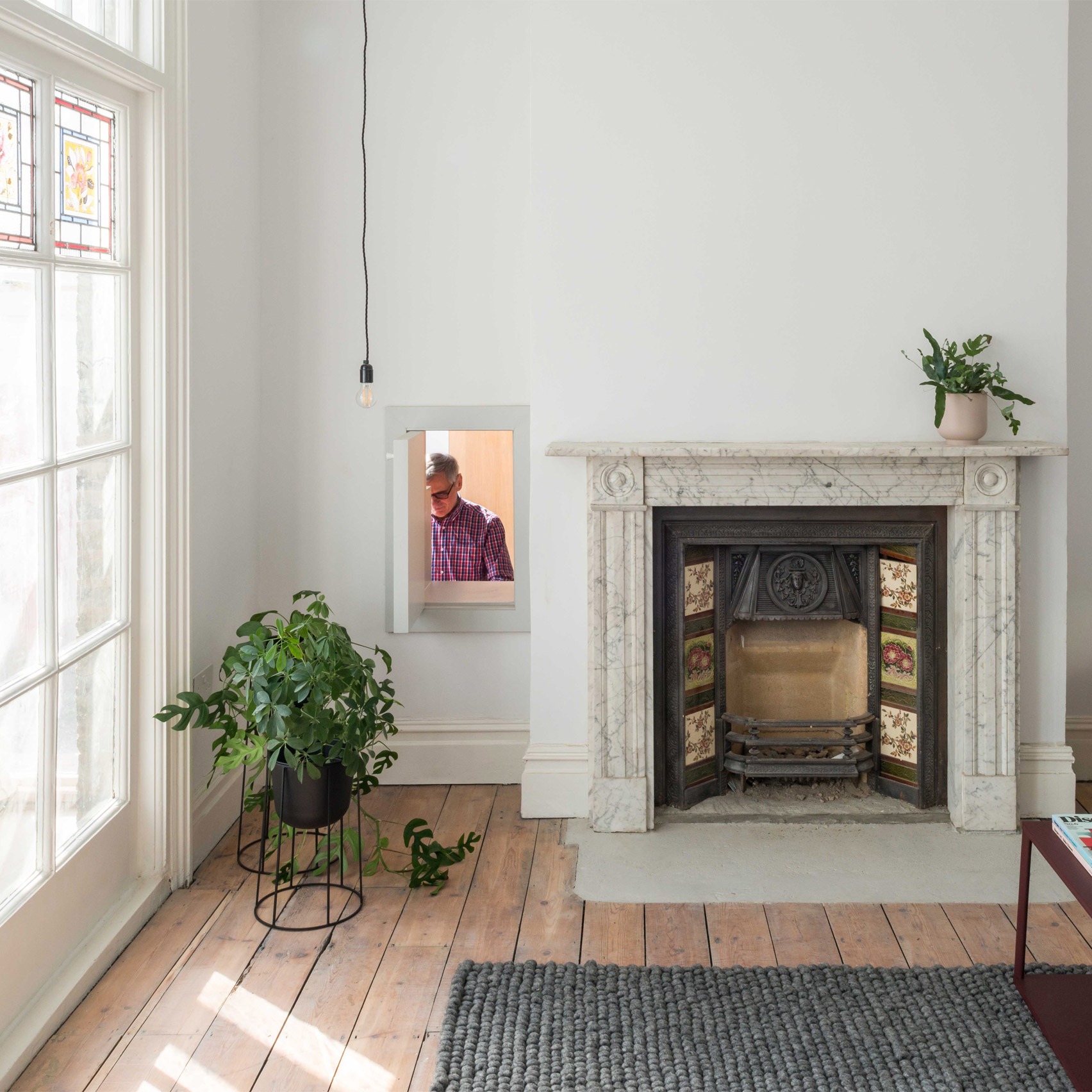This photograph depicts a beautifully detailed living room with a touch of both rustic and historic charm. The walls are painted white, creating a bright and airy atmosphere, further emphasized by a large floor-to-ceiling window on the left. This window, divided into eight panes, features a top row of stained glass adorned with a delicate flower design framed by a red line. Directly in front of the window, two green potted plants sit on raised black stands, their trailing leaves cascading elegantly onto the light brown, wooden plank floor.

Central to the room is a striking gray braided rug that anchors the space in front of a sophisticated fireplace. The hearth, flush with the floor, is gray, while the ornate mantle boasts a light gray marble finish with black veining, adding a touch of old-world elegance. The fireplace insert is a sleek black with a bronze border, and the interior of the firebox is a muted beige.

Flanking the fireplace on both sides are three square pictures, adding a symmetrical element to the decor. A small green plant in a pink planter sits on the right side of the mantel, injecting a subtle pop of color into the room. To the left of the fireplace, there's a windowed door that’s open, revealing a glimpse of another room with peach-colored walls. A gray-haired man wearing dark glasses and a maroon checkered shirt stands in this adjacent space, looking down, adding a curious narrative element to the scene.

The room also features a brown coffee table, partially visible, with a stack of magazines on it. At the center of the room, a long light string with a bare bulb hangs between the window and the fireplace, adding a simple yet industrial touch to the aesthetic. Overall, this living room exudes a blend of rustic charm and historic elegance, inviting a warm and intriguing ambiance.